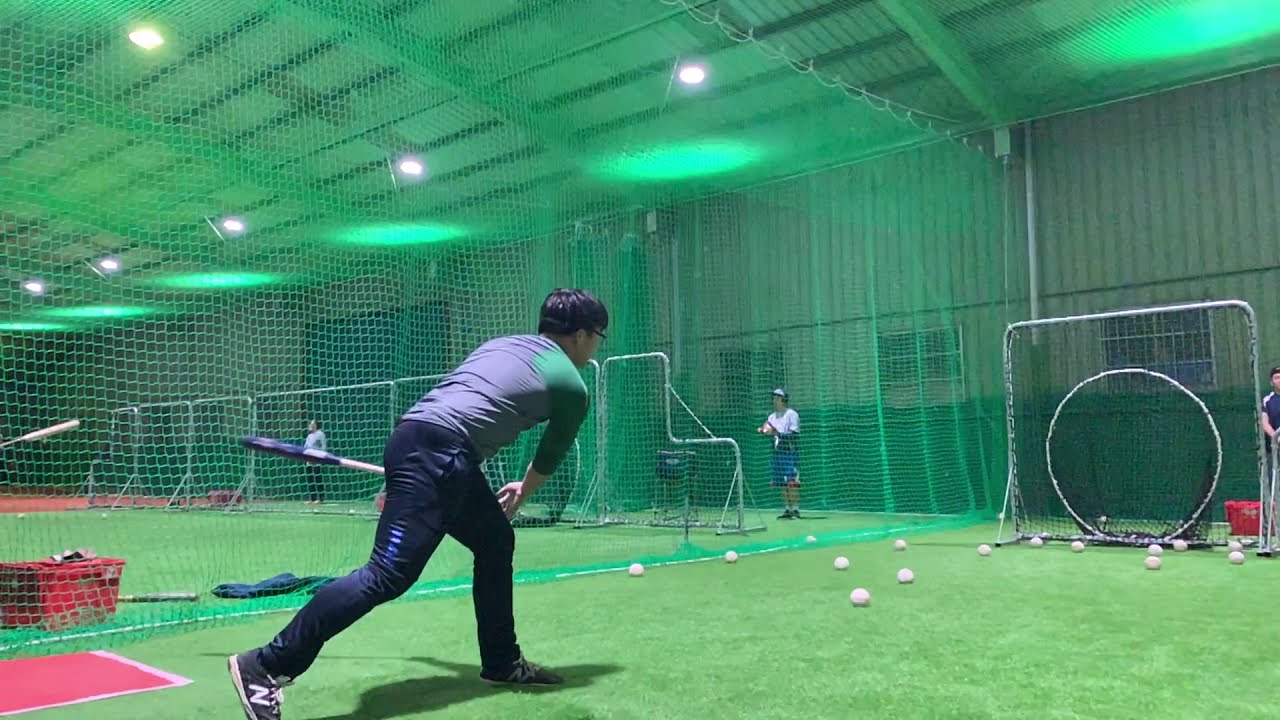This indoor photograph captures a bustling batting cage arena with a distinctly green hue, courtesy of the artificial turf covering the floor and the corrugated metal walls and ceiling. The space is divided into multiple rows—about four to eight—separated by mesh fences and netting, creating individual practice areas. In the foreground, a man of Asian descent in a purple and green shirt, black pants, and New Balance shoes is mid-follow-through from a swing. He is positioned near a unique net with a square frame and a circular target in the center, specifically designed to catch hit balls.

Adjacent to him is another man preparing to pitch, dressed in a blue shirt with white stripes on the shoulders. The foreground is scattered with baseballs, evidence of the batting practice in progress. People in helmets can be seen in the background, and other individuals are engaged in both pitching and hitting within their respective cages. The entire scene is enveloped in a framework of thick beams supporting the netted ceiling, encapsulating the environment's purpose and functionality.